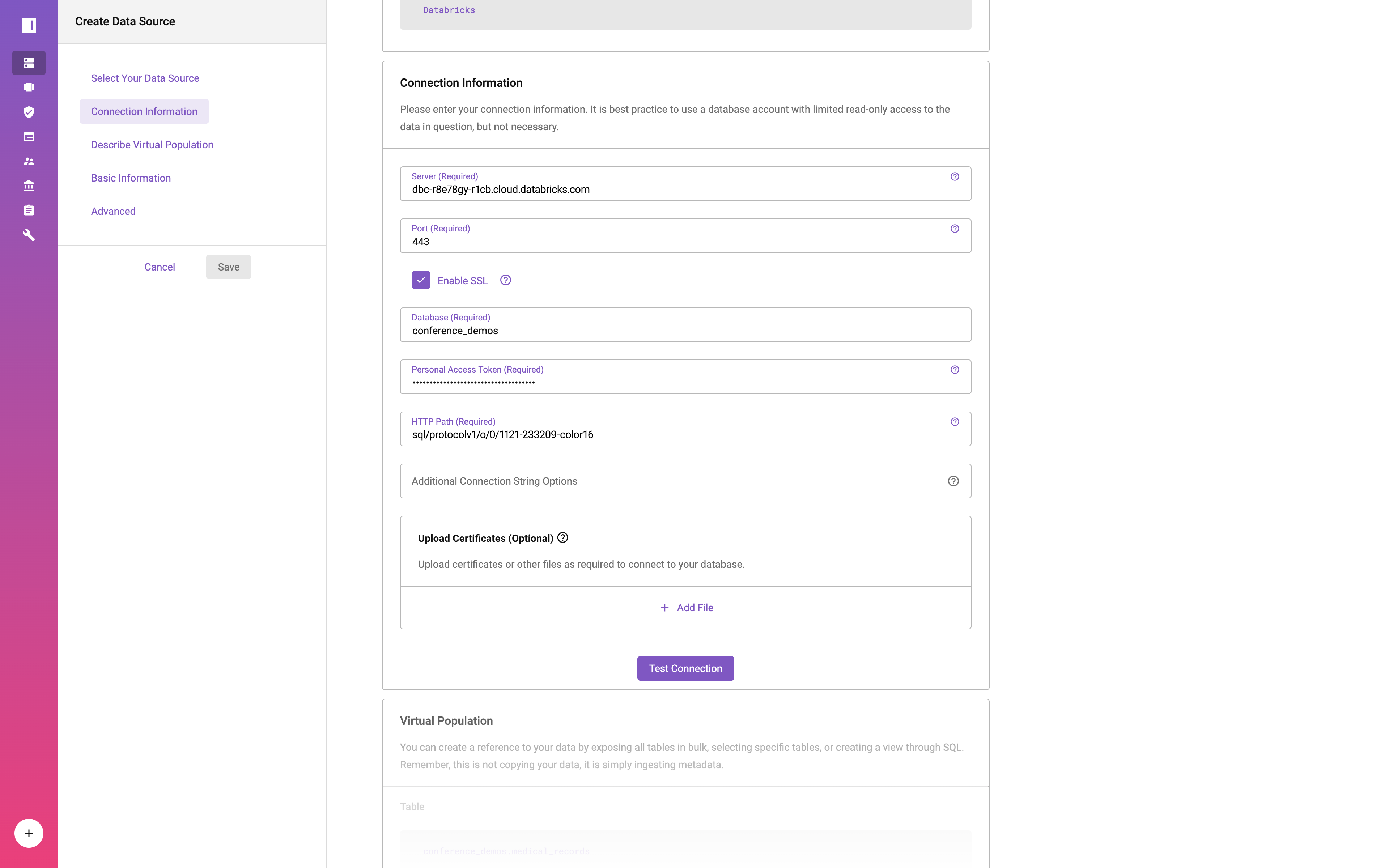The image consists of two vertical rectangular sections placed side-by-side on a white background. The left section is narrower and features a visually striking design element, while the right section is wider with a simpler layout.

**Left Section (Narrower):**

- **Background:** White.
- **Visual Element:** A vertical gradient ribbon on the left side, transitioning from blue at the top to pink at the bottom.
- **Top Banner:** A light gray ribbon with the text "Create Data Source" in black.
- **Vertical Ribbon Content:** Several icons representing different activities.
- **Lower Content:** Beneath the light gray banner, the white background displays gray text reading "Select your data source."
  - **Subsections:**
    - A gray box labeled "Connection Information."
    - Subsequent gray-text labels: "Describe Virtual Population," "Basic Information," and "Advanced."
- **Divider:** A thin gray line.
- **Action Buttons:** At the bottom, a gray "Cancel" button on the left, and a gray "Save" button on the right.

**Right Section (Wider):**

- **Background:** White.
- **Top Text:** "Connection Information" in black.
- **Subtext:** Gray text instructing users to enter their connection information. It advises that using a database account with limited read-only access is best practice.
- **Connection Fields:**
  - A long white text box containing a string of numbers and letters followed by ".cloud.databricks.com."
  - Below it, a white box labeled "Port" with the number "443" inside.

This detailed layout provides a clear and comprehensive visual description of the elements present in the image, aiding in user interface understanding and functionality.